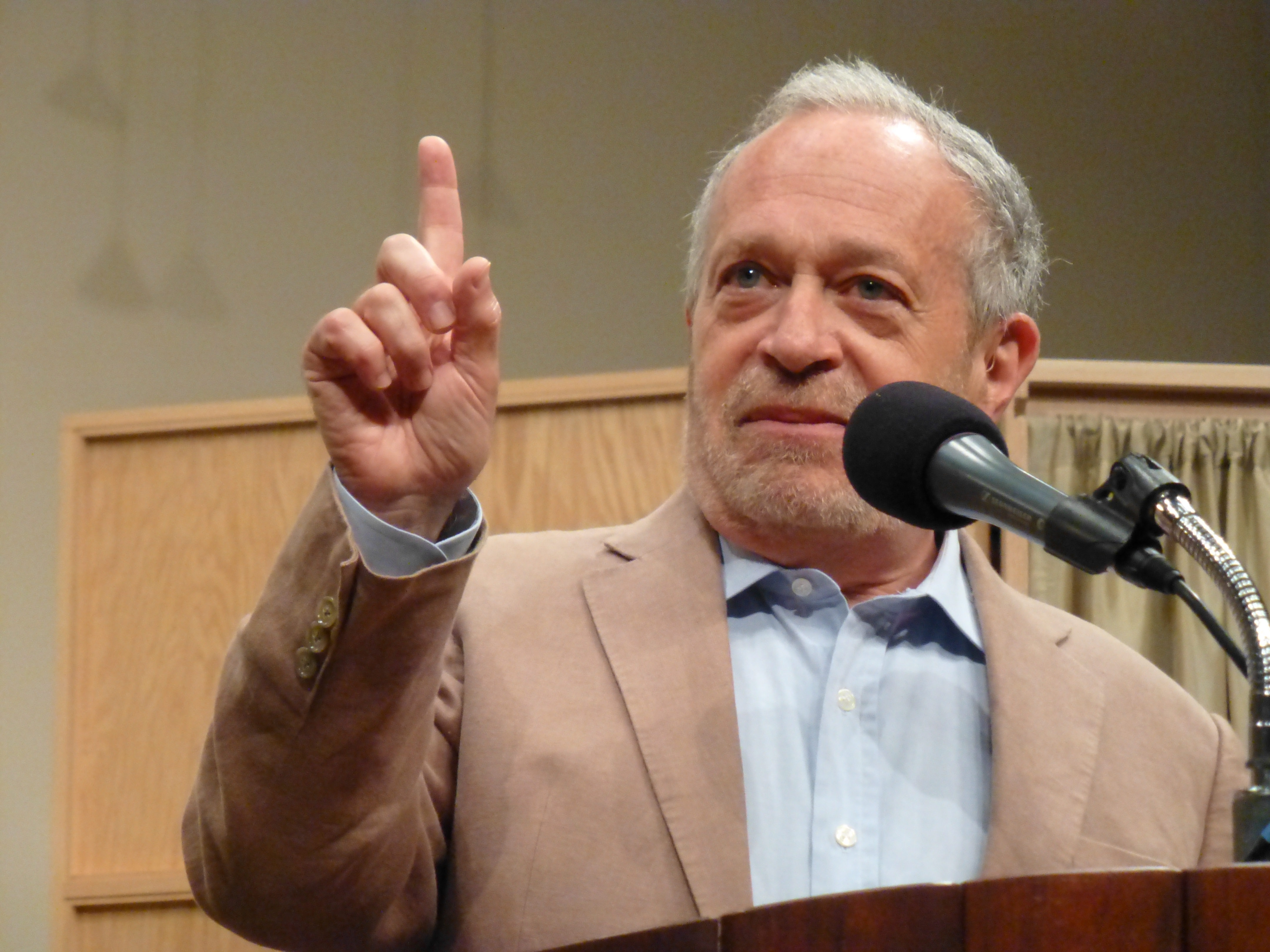The image depicts Robert Reich standing behind a wooden podium equipped with a metal stand and a plastic clip securing a black microphone. Reich, attired in a tan suit and a blue button-up shirt, raises his right hand with his index finger extended, as if making a point. His short, gray hair and a light mustache and beard frame his face. He gazes slightly to the left. Behind him, various elements populate the background, including a light green curtain to the right, brown furniture, and a booth-like wooden structure. Shadows from lighting create a white backdrop, adding depth to the scene.